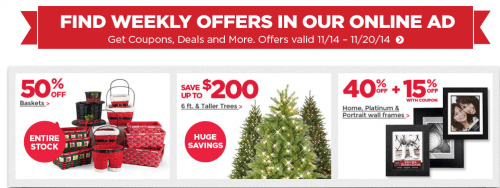This page showcases a variety of prize offerings, displayed across three distinct images representing different categories. Each section features enticing shopping baskets and hampers brimming with goodies, alongside beautifully decorated Christmas trees that add a festive touch. Framing the images are elegant picture frames that enhance the visual appeal. The accompanying text highlights the promotional details, stating: "Find weekly offers in our online ad. Get coupons, deals, and more. Offer valid from 11-14 to 11-20."